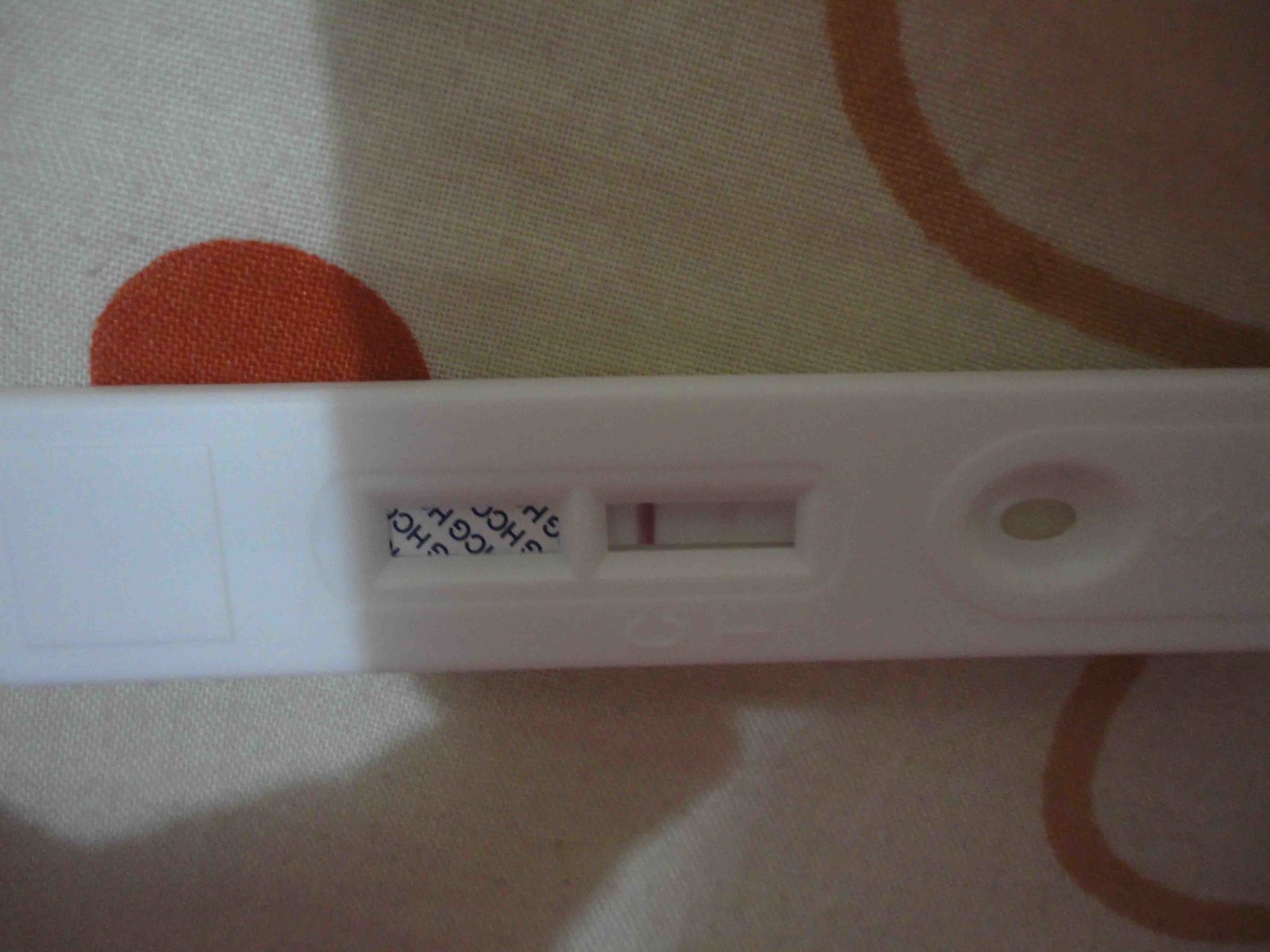The photograph features a real-life setting with a felt background, prominently in a vibrant red color. Centered on this background is a white rectangular stick, resembling either a pregnancy test or a COVID test. The stick is placed horizontally, stretching from the left to the right of the frame. It displays two distinct markings: a red stripe next to the letter "C" and several blue letters in an adjacent box that spell "HCG." This suggests the test is likely a pregnancy test, given the reference to HCG (a hormone produced during pregnancy). The red stripe indicates a positive result on this test. The overall composition emphasizes the test device, making it the focal point against the contrasting red felt background.